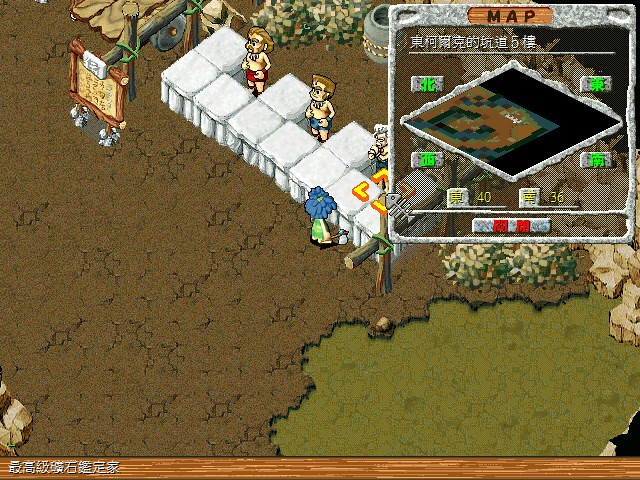This is a detailed screenshot from a video game set in a caveman era. The majority of the left side features a brown dirt terrain that stretches diagonally from the lower left to the top right. As you move towards the upper right corner, a line of white squares becomes visible, resembling large boulders. Standing within these squares are three caveman-like figures, wearing loincloths and necklaces made from what appear to be stone or saber tooth tiger teeth. 

In the top right corner of the image, a map area is depicted, bordered by a gray outline. Inside this map, there are Japanese or Chinese writings, a diamond shape, and a small rectangular section showing water and land features. To the bottom right is a green patch, indicating a grassy area.

The lower left corner contains white writing in Japanese or Chinese on a wooden beam-like banner stretching across the bottom of the image. The cavemen are detailed with the first having long hair, red shorts, and a mustache. The second, positioned down and to the right, has blue shorts and brown hair. The third man, further down and to the right, has gray hair and blue shorts. Opposite them, across the white blocks, stands another figure in a green dress with a large blue hairdo, holding an axe. Additionally, a small wooden structure with signage is visible to the top left.